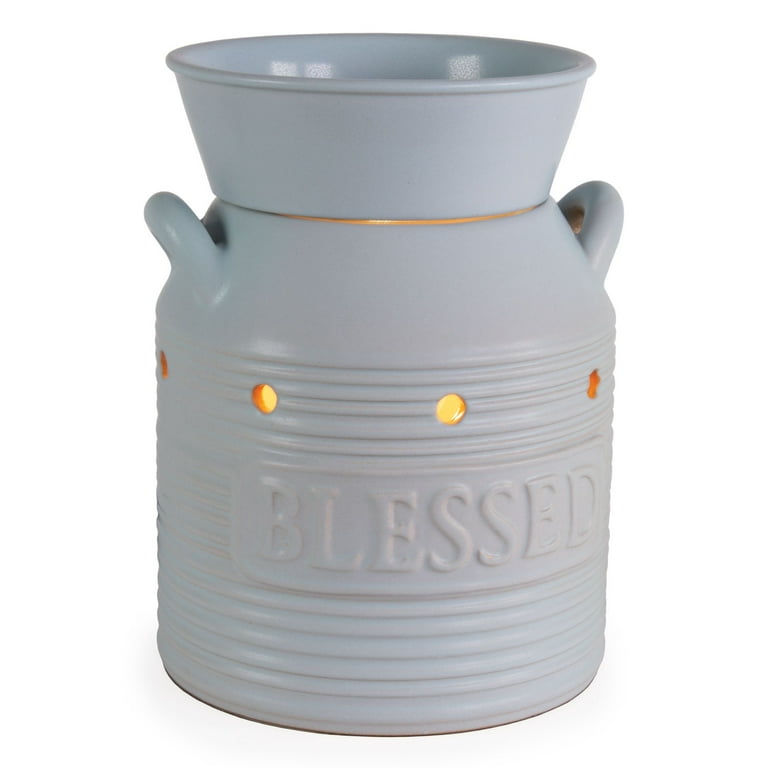This image showcases a detailed, up-close photograph of a blue ceramic candle holder or wax warmer designed with two small handles on either side. The jar-like shape is reminiscent of a milk canister, with a ridged pattern running along the bottom part of the holder. Light from what appears to be a candle or potentially a light bulb creates a flickering yellow-orange glow that shines through small circular holes scattered across the surface, including below the handles. The top of the holder, which appears to house the candle or wax melts, allows a bit of light to escape as well. Prominently embossed in the solid, smooth area above the ridges, the word "Blessed" is rendered in the same blue color, adding a touch of sentimental charm to the piece.